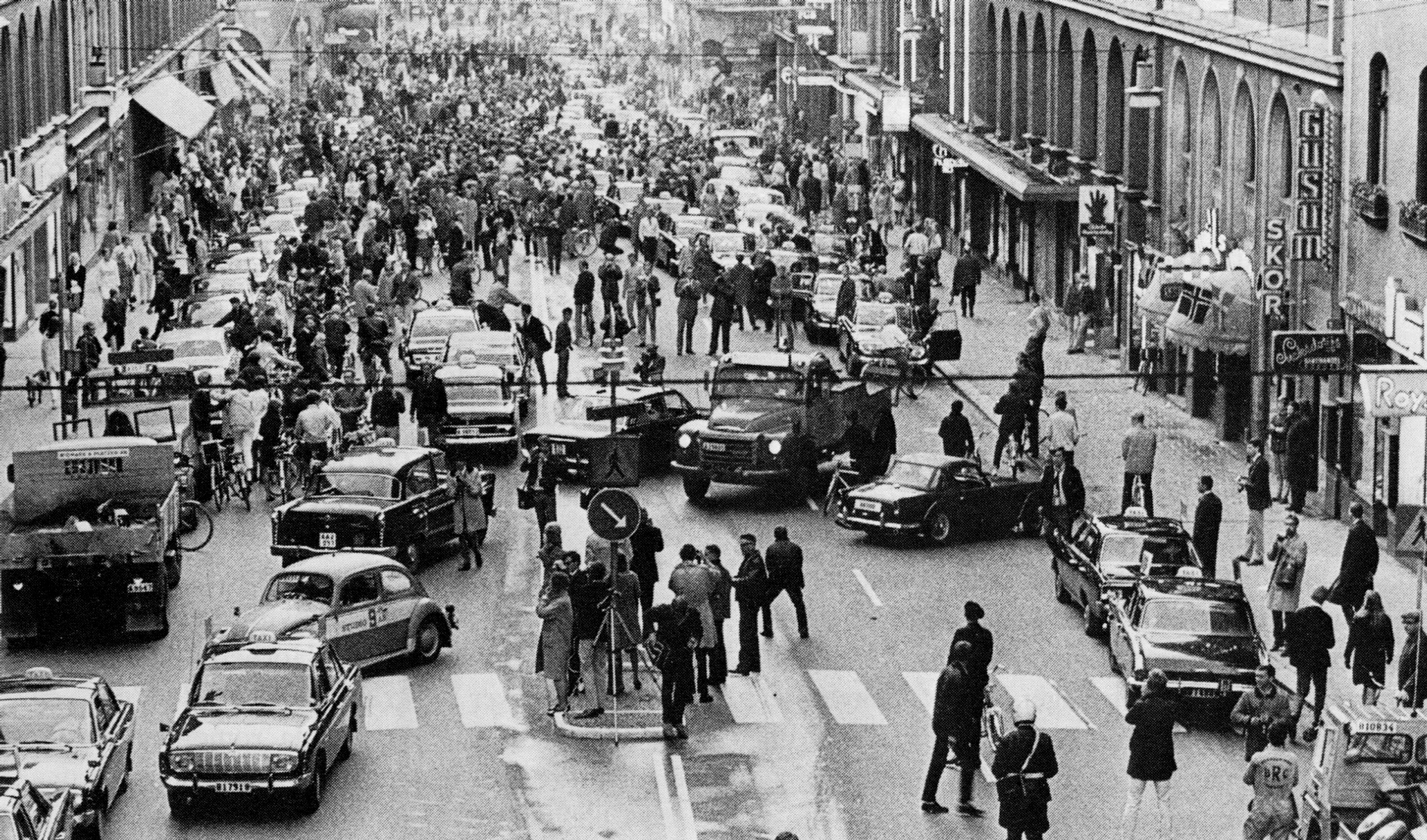This iconic photograph captures the historic moment in the 1960s when Sweden transitioned from driving on the left side of the road to driving on the right, an event known as "Dagen H" or "H Day." Set in a bustling downtown area, the overhead view vividly illustrates the confusion that ensued among both drivers and pedestrians. The image showcases a crowded city street, with cars halted and pedestrians stranded in the middle of crosswalks, visibly perplexed by the abrupt change. People conditioned to look for traffic coming from one direction are now bewildered as they adjust to the opposite flow. Vehicles are seen backed up, highlighting the widespread disruption caused by this significant switch. The photograph stands as a testament to the profound psychological and logistical challenges faced during this monumental transition in Swedish urban life.